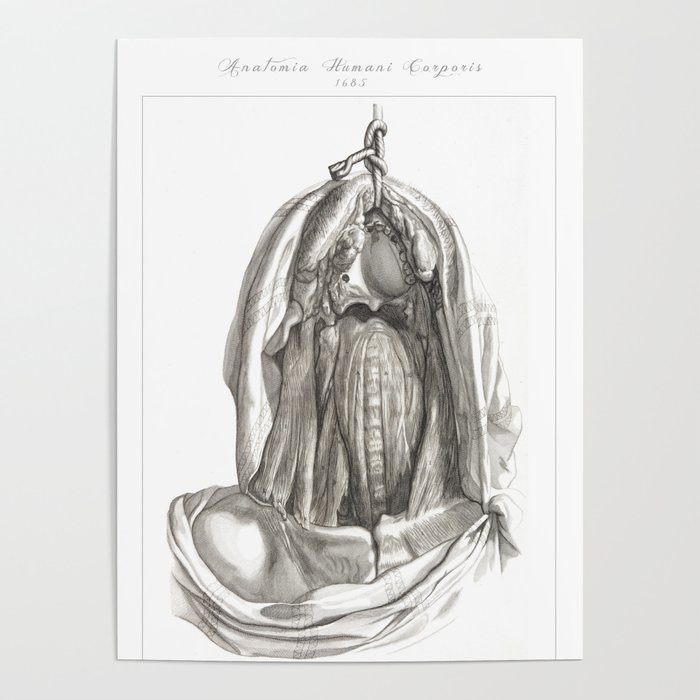This is a large square picture of a poster on a light gray wall, featuring a vertical rectangle with a detailed sketch. At the top, it reads "Anatomia Humani Corporis, 1685" in a cursive font. The sketch is framed by a thin black border and appears to depict an anatomical illustration, blending elements of internal human anatomy with a gown. A bar with a rope or string wrapped around it suspends the illustration, creating an impression that the anatomical features are hanging. The drawing, executed in brown and white tones, shows what resembles internal organs rather than bones, with parts of the gown draped and angled outward, particularly towards the left at the bottom. The ambiguous mix of anatomical parts and clothing creates an intricate yet perplexing image, suggesting a historical approach to human anatomy representation.